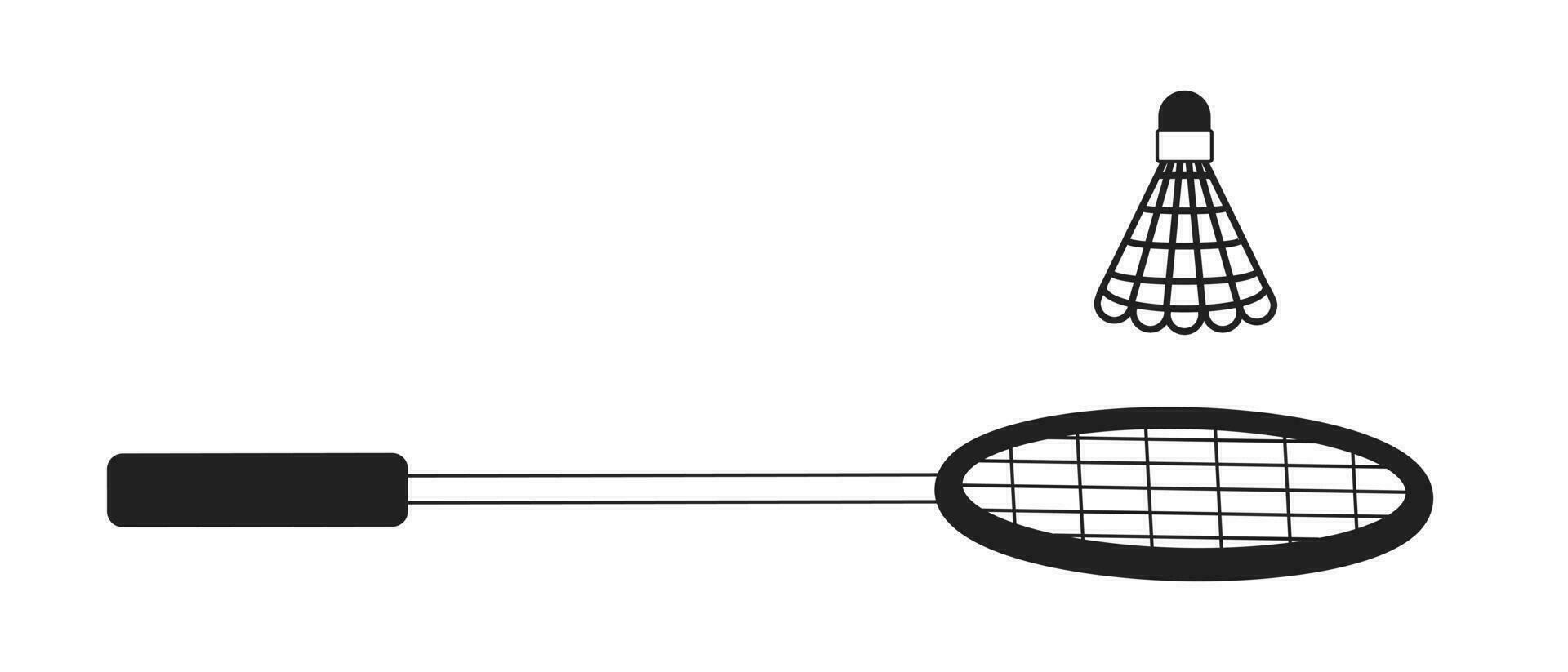This image features a detailed, computer-generated black-and-white line art illustration set against a white background. Central to the composition are a badminton racket and a shuttlecock. The racket is positioned horizontally across the lower part of the image, with its solid black handle extending from the left. The handle transitions into a black-outlined shaft that connects to the racket's elliptical face on the right. The face of the racket is depicted with a solid black border encompassing a mesh grid pattern, indicating the stringed hitting surface.

Above the racket floats the shuttlecock, oriented with its rounded, solid black rubber tip pointing upwards. The fan-shaped lower portion of the shuttlecock, rendered in a delicate black outline, represents its mesh structure. This portion fans out in a scalloped pattern, indicative of its intricate design. The mesh gradient below the tip creates a sense of depth and texture to the feathers, which are actually plastic. Overall, the illustration captures the essence of these badminton equipment pieces in a minimalist yet highly descriptive style, without any additional elements or borders.